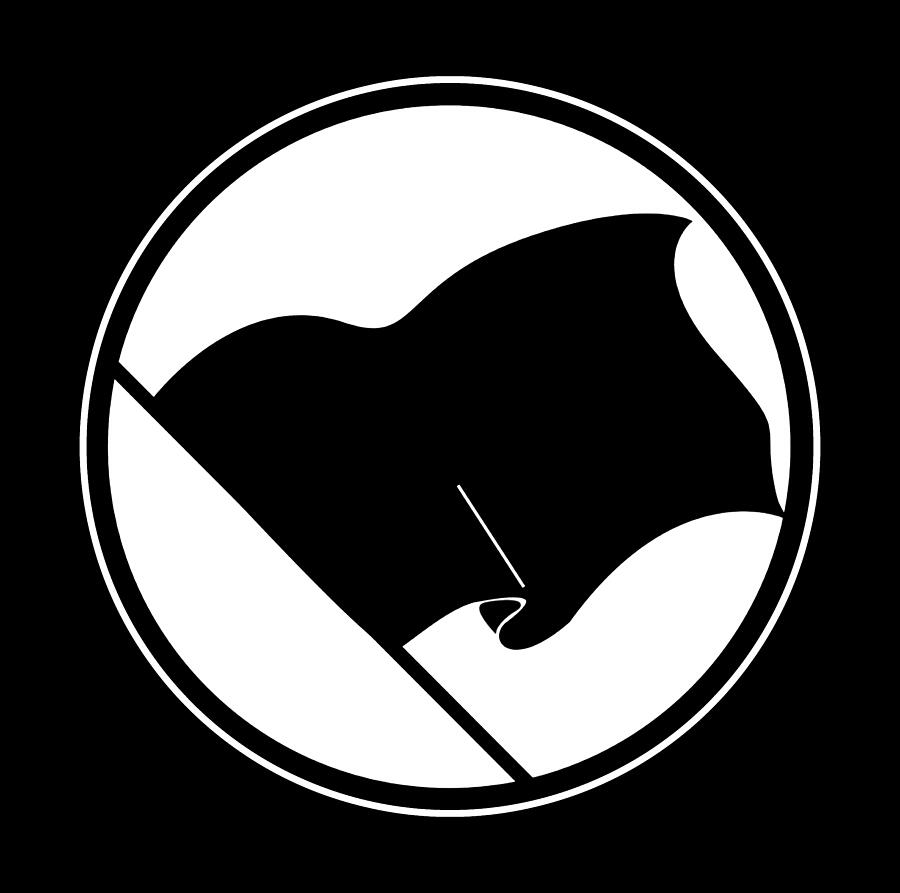The illustration features a black square as a background. Centered within this black square is a white circle, meticulously outlined with a thin white border, followed by a slightly thicker black border. Inside the white circle, a black flag dominates the scene, resembling a silhouette painted entirely in black. The flag appears animated, waving gently as if moved by a subtle breeze, enhancing its dynamic presence. A flagpole on the left side extends from the bottom middle of the circle to the upper left part, firmly anchoring the flag. Intriguingly, a white line is visible near the bottom of the flag, following the contours of its ripples and extending about halfway up, adding to the depth and detail of the portrayal.